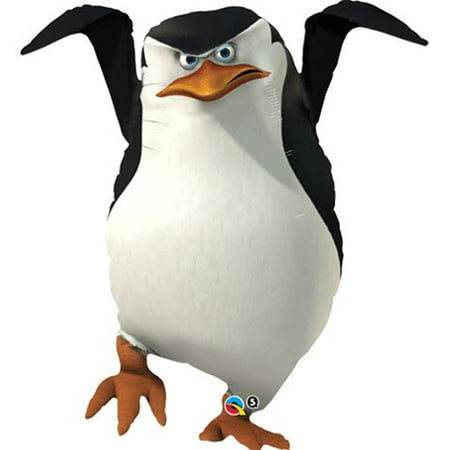This is an illustration of a cartoon penguin, reminiscent of a character from the Angry Birds collection, set against a plain white background. The penguin features the classic black and white coloration: a white belly and face complemented by a black head. Its eyes are notably expressive, with white sclera and black pupils, highlighted by a subtle blue tint. The beak and feet are a reddish-brown, with the feet depicted as three-fingered. The penguin strikes a defiant pose, with wings extended upward and a stern expression enhanced by a furrowed brow. Its right leg is lifted, reminiscent of a stance from Cobra Kai, while the left leg remains firmly planted on the ground. Notably, the left ankle appears adorned with a bracelet-like detail featuring a blue top, a red bottom, and a yellow streak, accompanied by another black circle with a white 'S' just to its right.